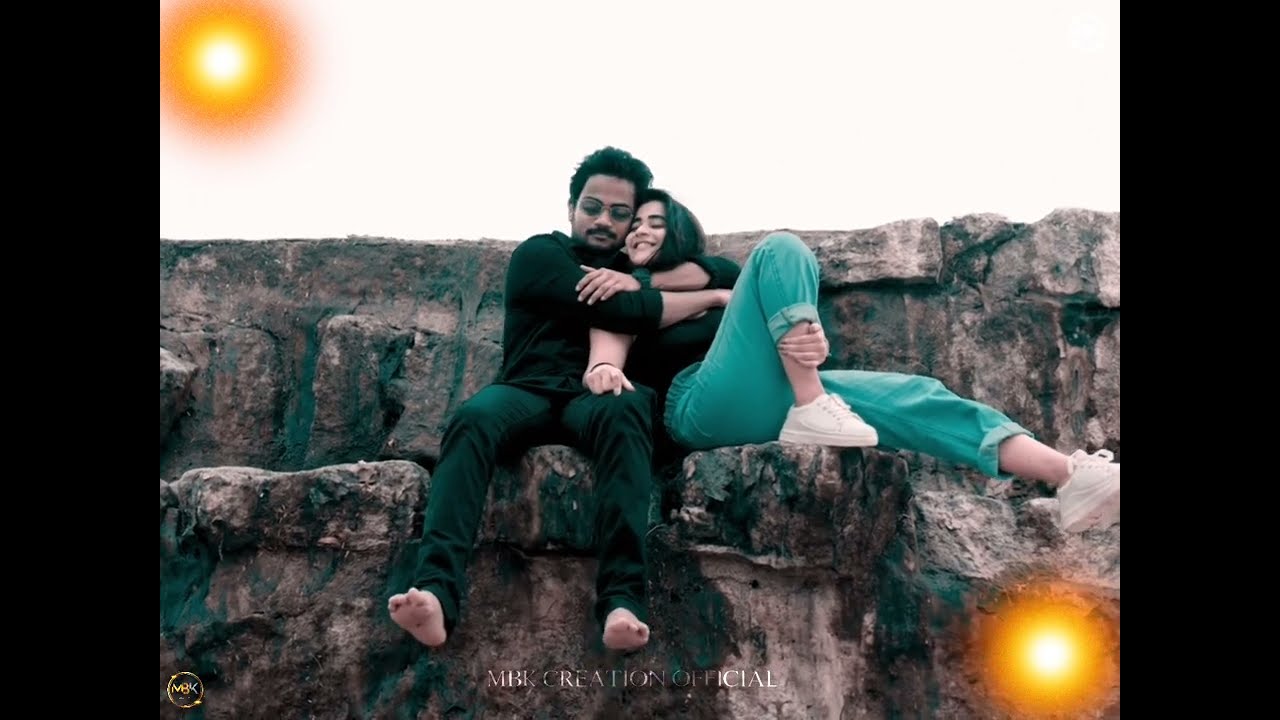The image depicts a couple seated on the ledge of a stone structure, with two black vertical bars framing the left and right edges. The stone structure is composed of medium-brown rectangular blocks, heavily covered in dark green moss. The couple occupies the center of the image, seated on the bottom third of the frame. Above them stretches another horizontal stone ledge, indicating an intentional architectural design. 

The man, positioned on the left, is barefoot and dressed in long black pants and a long black sweater with sleeves rolled up to his elbows. He has short black hair, a mustache, and glasses, and his complexion suggests he might be of Indian descent. His arms are wrapped protectively around the woman beside him. The woman, on the right, has long black hair and a similarly darker skin tone. She wears a black top, light green pants, and white tennis shoes, her right arm resting on his lap as she leans into him.

In the background, the sky is a uniform white with no distinguishable sun or stars. However, lens flares, or balls of orange light, are visible in the upper left and bottom right corners of the image. At the very bottom of the photograph, a translucent, white text reads "MBK Creation Official," with a similar golden circle bearing the initials "MBK" in the bottom left corner.

This image, likely the work of a professional photographer, captures an intimate moment between the couple against the backdrop of an artfully designed stone structure.